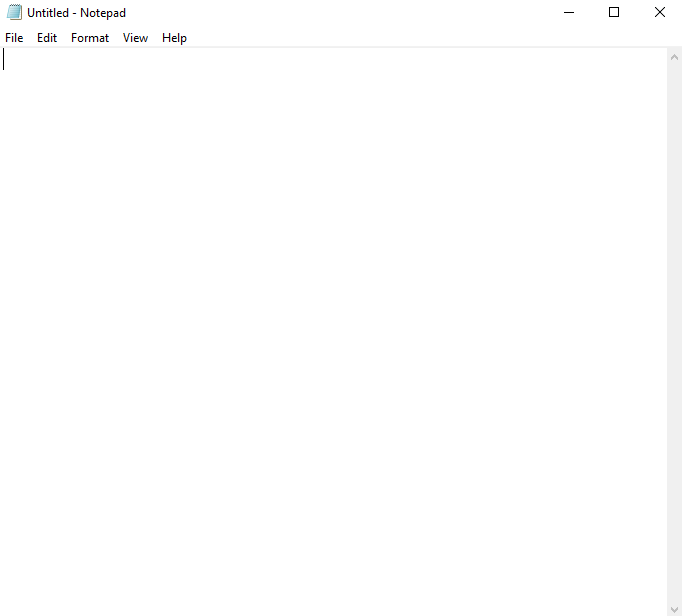The image depicts a blank Notepad window on a computer screen. At the very top left, there is a Notepad application icon featuring a blue sheet of paper slightly flipped to reveal additional sheets beneath. Next to the icon, the title "Untitled - Notepad" is displayed, with both "Untitled" and "Notepad" starting with capital letters. Below the title bar, the menu options "File," "Edit," "Format," "View," and "Help" are listed, each with their initial letter capitalized.

The main body of the Notepad window is a blank, white page, awaiting text input. A thin vertical line indicates the starting point for entering text. On the right side of the window, there is a grayed-out vertical scroll bar, signifying that there is no content to scroll through. The scroll bar features an arrow at the top and an arrow at the bottom for navigating up or down once text is entered. Overall, the image portrays an untouched Notepad document ready for use.